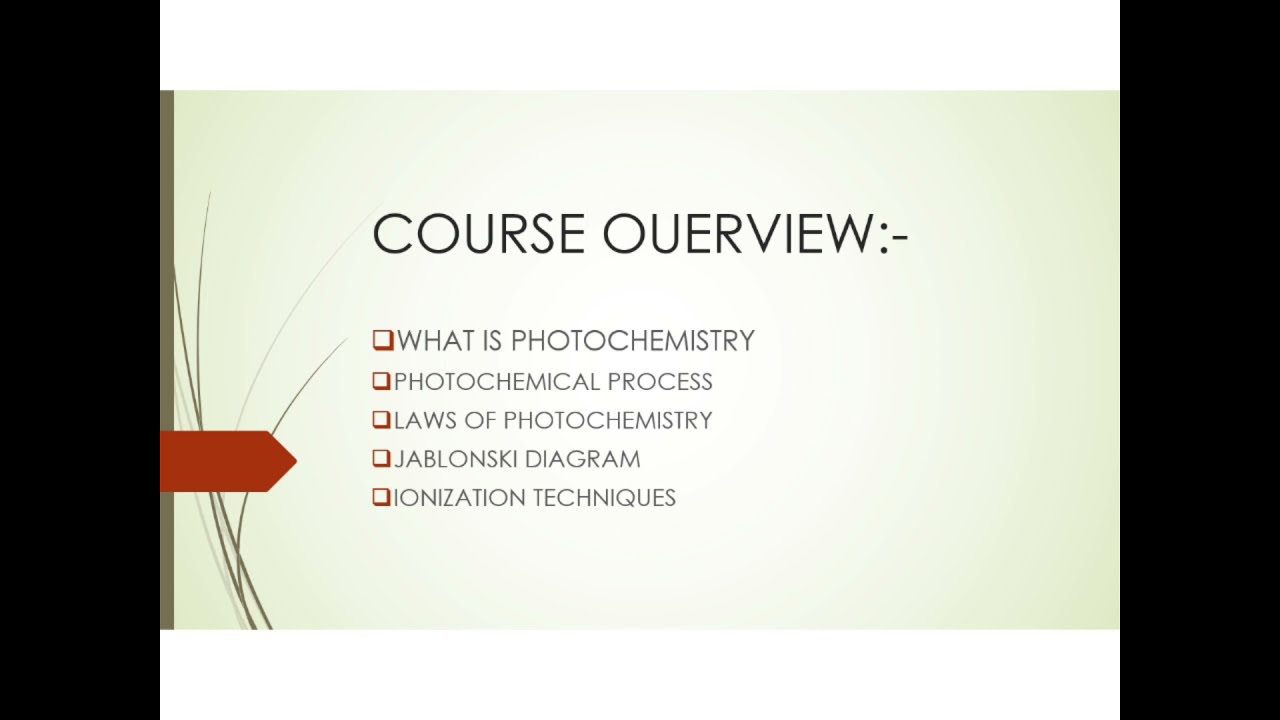The image is a wide rectangular screenshot of a PowerPoint slide, likely created in Microsoft PowerPoint, that forms part of a presentation. The slide features a light greenish-gray background that fades to lighter shades towards the center. At the top, in bold black font, it reads "Course Overview." Below this heading, five bullet points are listed: "What is Photochemistry," "Photochemical Process," "Laws of Photochemistry," "Jablonski Diagram," and "Ionization Techniques." Each bullet point is accompanied by a small red square box on its left.

On the left side of the slide, there is a thin vertical strip in a pea-green color with several wispy, curving lines extending upward from the bottom. Additionally, there is a burnt orange tab with an arrow pointing toward the right, directing attention to the bullet points. The slide is also bordered by black vertical bars on both the left and right sides. Horizontal white bars appear at the top and bottom borders of the slide, framing the content neatly. All elements in the image are properly oriented and upright.